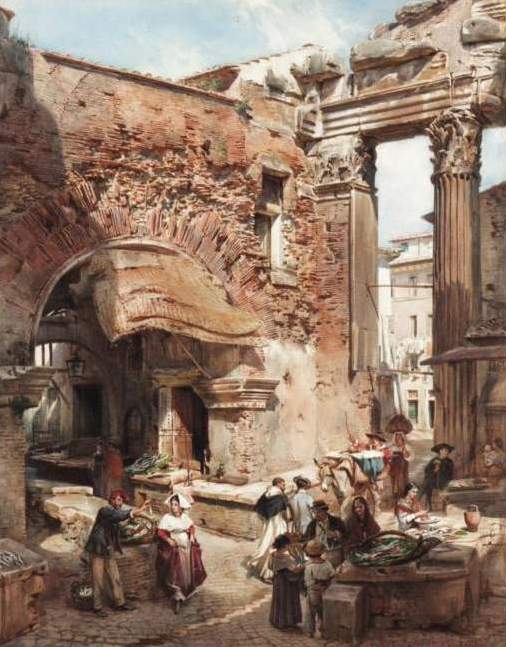The image depicts an intricately detailed, hyper-realistic painting of an ancient, possibly Roman or Greek, plaza. This vertically aligned rectangular image showcases a grand stone structure with an arched walkthrough area, partially covered by a built-in stone canopy. On the right side of the painting towers a massive marble column with vertical grooves, supporting another stone piece overhead. The structure appears aged, with reddish rust staining portions of the archway and signs of damage hinting at a tumultuous past.

In the foreground, a bustling market scene unfolds, populated by men, women, and children all dressed in period-appropriate attire including long gowns, dresses, headdresses, and a man wearing a tricorn hat. On the left, a man in brown pants and a blue shirt stands next to a woman in a white and red dress, gesturing animatedly. To the right, more figures gather around a stone table on which rests a jug and a coiled object. The plaza is alive with activity, highlighting the various shades of black, white, gray, brown, tan, red, green, and coppery hues that dominate the scene. In the background, additional ancient structures loom, enhancing the authenticity and historical depth of the painting. The sky above is a clear blue with feathery white clouds, adding a touch of tranquility to the otherwise dynamic scene. A donkey makes its way through the space between the column and the wall, further emphasizing the lively, everyday market atmosphere of this ancient courtyard.